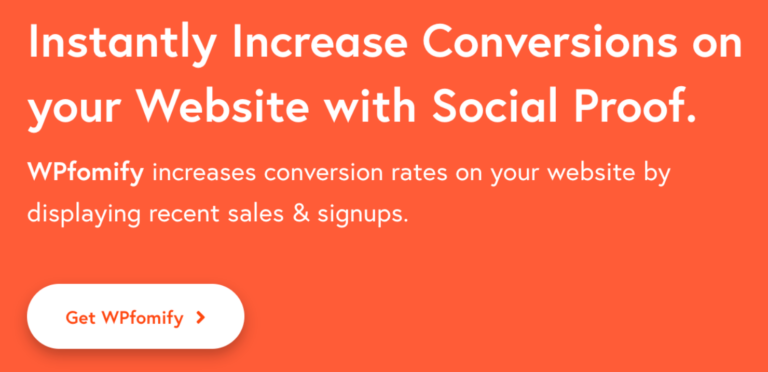The image features an orange background with prominent white text. At the top, in a larger, bold font, it states, "Instantly increase conversations on your website with social proof." Below this, in a slightly smaller, yet still white font, it reads, "WP Phone 5 increases conversation rates on your website by displaying recent sales and signups." To the left side, the text continues with "Get WP Phone 5," accompanied by an arrow pointing to the right. This section is enclosed in a white box, emphasizing the call to action.